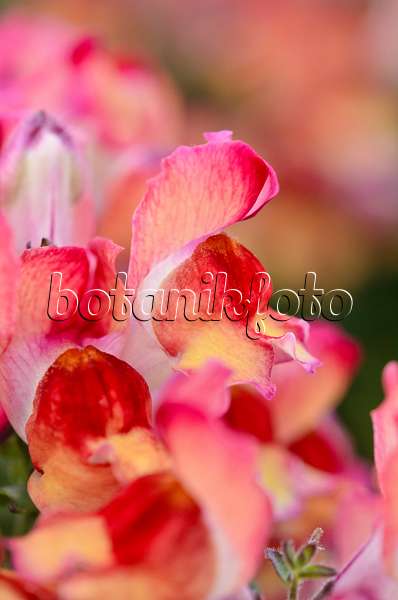This close-up outdoor photograph captures a vibrant array of flowers with delicate petals. The image is mostly composed of pink and red flowers with intricate details that gradually become blurry towards the edges. The top half of the photograph, extending from the upper left corner to the upper right, is noticeably blurred, making it difficult to distinguish specific details but hinting at more flowers in hues of yellow, pink, and green in the background. The bottom part shows additional flowers and some green leaves or branches on the left side. Across the center of the image, there is a semi-transparent watermark that reads "BOTANIK FOTO" in a clear yet thick, bubble-like font with a black border, adding an artistic touch to the photograph's overall serene and colorful aesthetic.